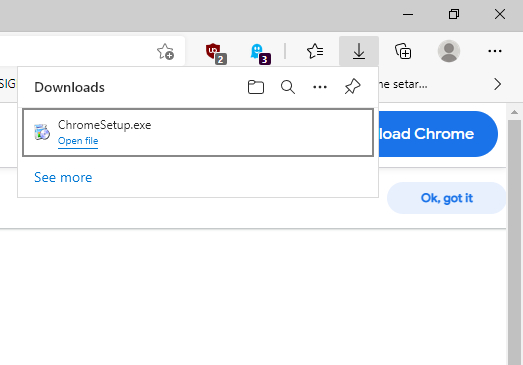Screenshot of a download prompt within a web browser interface. At the top of the window, a gray bar contains various icons including a red 'X' for closing, a double square for duplicating, a star for adding to favorites, and a shield with the number "2" indicating security features. Adjacent icons include a ghost with the number "3", a star with horizontal lines signifying bookmarks, and a downward arrow alongside a copy icon and a person icon representing user profiles.

Beneath this toolbar, the section is titled "Downloads", presenting several options: a file icon, a magnifying glass for search functionality, three vertical dots for additional menu options, and a pen for editing. The text "ChromeSetup.exe" is displayed prominently with "Open file" in blue, suggesting an active link. Below this, "See more" and a blue "Download Chrome" button are visible, encouraging users to proceed with the download.

A dark gray scroll bar is located on the right side of the window. Towards the bottom, a light blue bubble contains the text "Okay, got it" in dark blue, offering an acknowledgment option. A gray dividing line separates this from partially cut-off text below, which is illegible. The overall layout is typical for browser-based download prompts, focused on usability and accessibility.